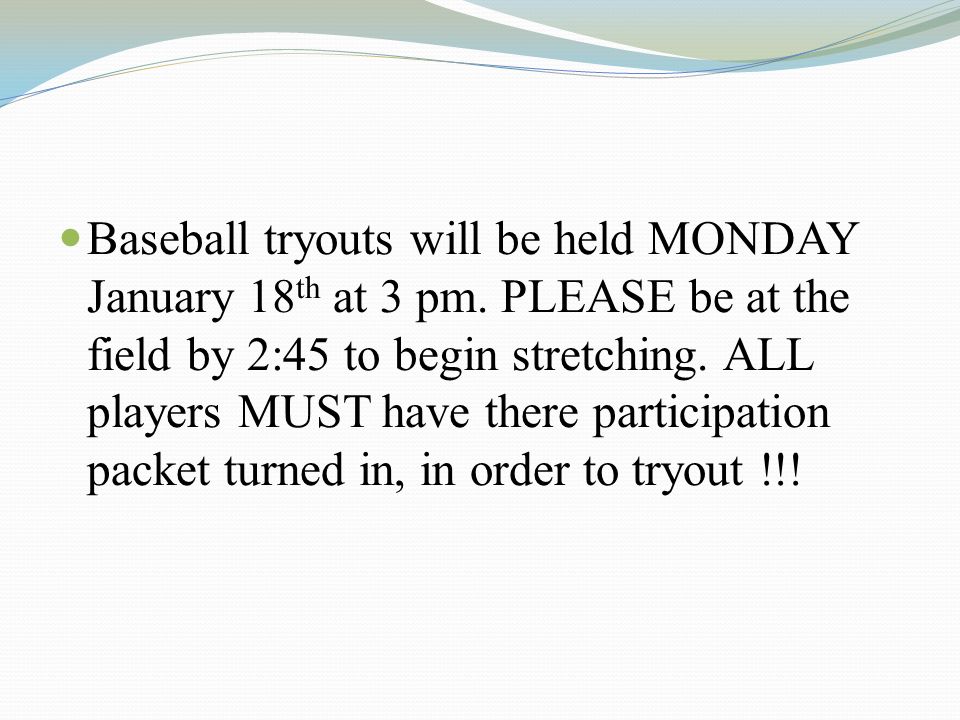The image is a PowerPoint slide with a predominantly white background. At the top, there is a wavy, bluish-greenish-gray pattern extending from the upper left to the upper right. Central to the image are five lines of black text, each line left-justified and beginning with a small green bullet point. The text details:

- Baseball tryouts will be held Monday, January 18th at 3 p.m. (The word "Monday" is capitalized.)
- Please be at the field by 2:45 to begin stretching. ("Please" is capitalized.)
- All players must have their participation packet turned in to try out. ("All" and "must" are capitalized.)

The slide has a minor typo where "their" is misspelled as "there," and it includes three exclamation points at the end. The style and layout suggest it is intended for distribution to sports team members or their parents, possibly as an announcement in warm climates since January is listed for the baseball event.